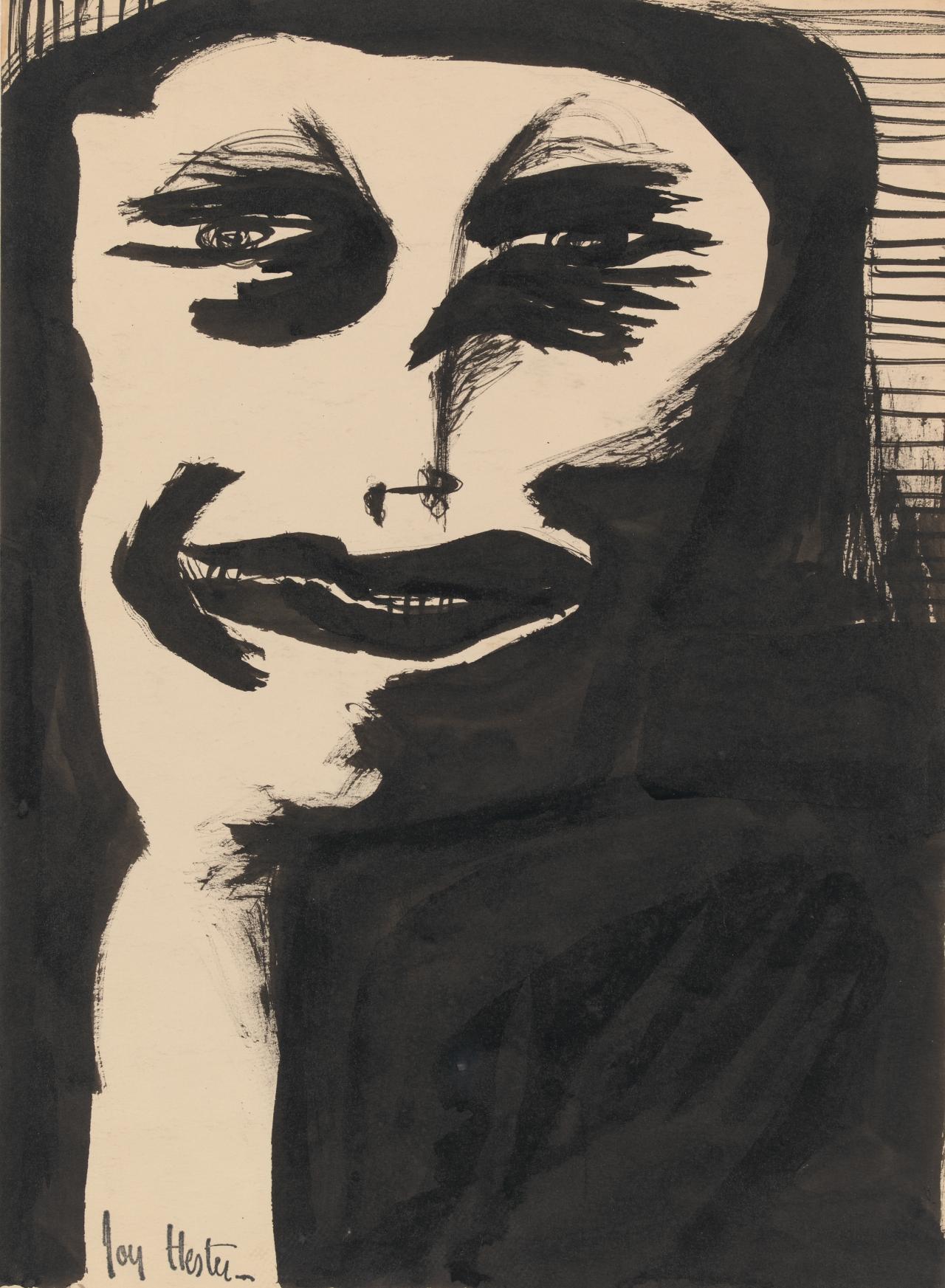This striking black-and-white artwork by Joy Hester features a large, central portrait of a person with distinct comic-book style qualities. The figure, which dominates the image, appears to be a woman. She is characterized by dark black lipstick, shaded eyes, large lips, and long black hair that cascades down, with the image cutting off at the top of her torso. The person has a very straight nose and a slightly crooked smile, adding to her unique look. There is a distinctive black arrow mark on the right side of her face. The background includes what appears to be a striped design or window blinds. The additional coloration is primarily in shades of black, white, and cream, with some suggestions of light brown. Below, at the bottom of the artwork, is the artist's signature, attributed to Joy Hester. The overall look is reminiscent of both comic book art and low-quality personal sketches.